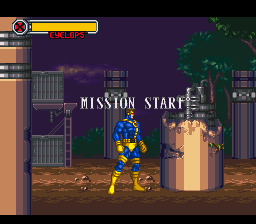This image, a square-sized screenshot from an old side-scrolling video game, features a dim, industrial scene reminiscent of a carnival at night. Centered on the screen are the words "Mission Start" in white letters. Dominating the middle ground is a massive, golden column that has a mechanical appearance, with its top apparently torn off to reveal what looks like a hand grenade inside. A figure, resembling a superhero, stands beside this column; he is extremely muscular, clad in a blue bodysuit with golden details, including gloves, boots, and a belt-like armor around his waist. The background is industrial, with metal silos that might be holding chemicals or acting as supports for separate structures. In the top left corner of the screen, a life bar appears fully filled in yellow with the name "Cyclops" written underneath in red letters. Adjacent to the bar, there is a red circle with a black X in the center, adding to the scene's dramatic and action-packed ambiance.